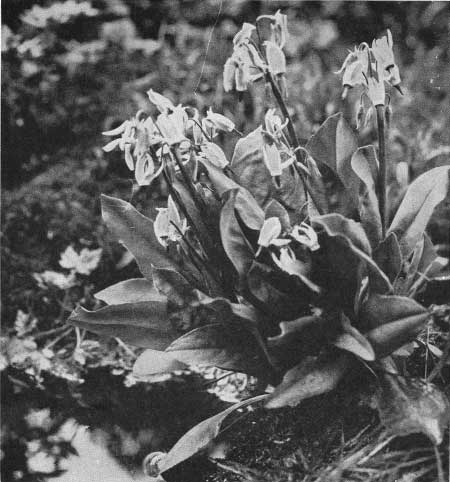This black and white photograph, likely of an older vintage and of low quality, depicts a clump of daffodils well past their prime, situated in a garden setting. The once vibrant flowers now hang limply from long stems, with many petals crinkled or already fallen to the ground, rendering them bare. The leaves, which are suggested to be green but indistinguishable due to the monochromatic nature of the photo, are prominently visible. The scene includes additional flora in the blurred background, enhancing the garden atmosphere. In the lower left corner, there appears to be a small pond reflecting the daffodils and surrounding plants, adding depth to the composition. Shadows of the withered flowers cast onto the ground contribute to the overall somber and nostalgic mood of this outdoor snapshot.